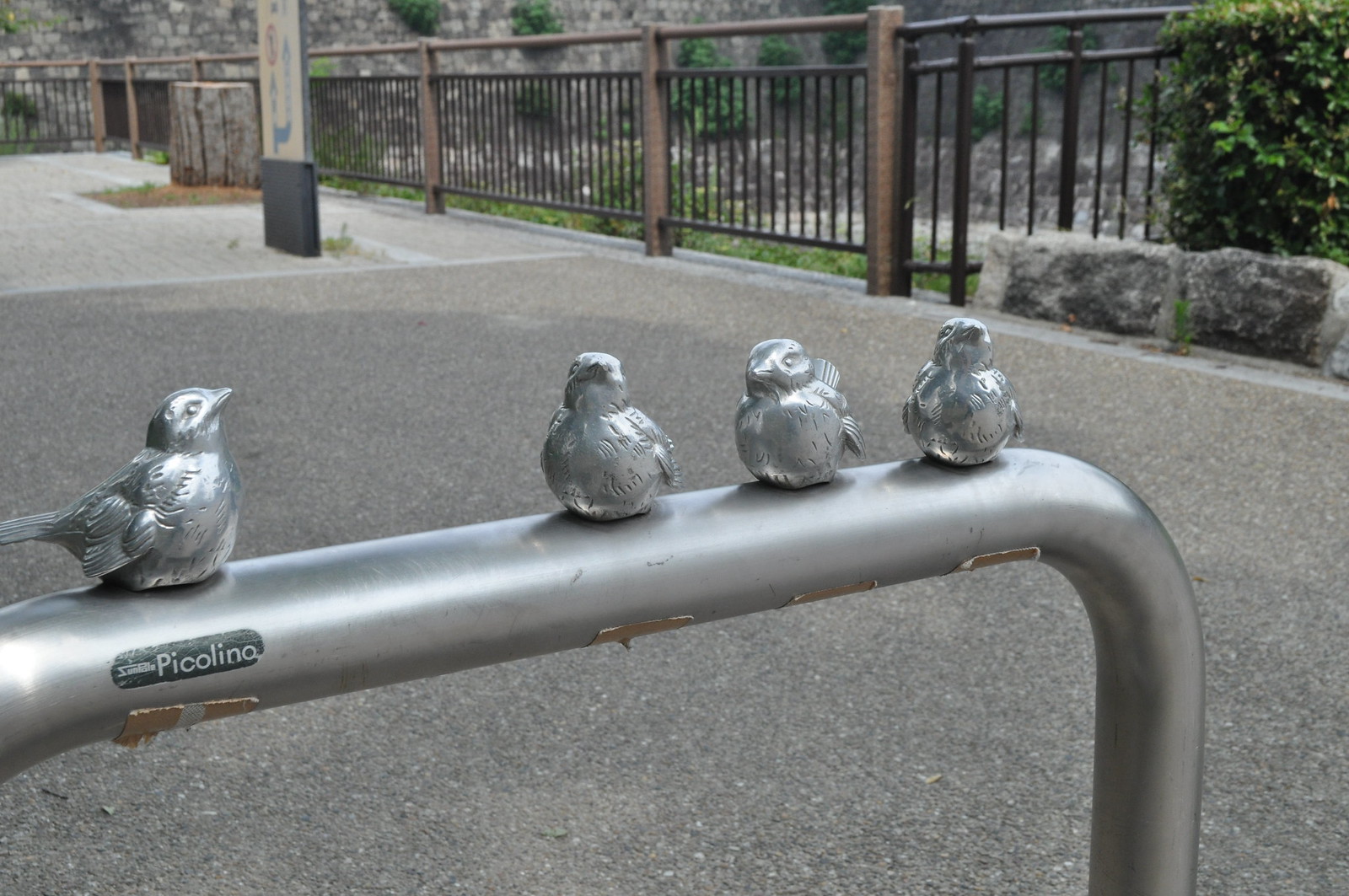This outdoor image captures a detailed scene centered around a grey, silver-colored pole adorned with four small, silver birds. These metallic birds, positioned facing forward with their beaks up, are spaced uniquely, with one bird on the far left and the other three clustered together towards the center. The pole, possibly metal, stretches diagonally from slightly above the lower left corner towards the right before bending downward. A black stripe encircles the pole with silver lettering that reads "Piccolo" and "Piccolino."

In the background, a brown and grey railing spans across the frame, featuring concrete pillars spaced evenly along its length. Behind this railing, parts of the setting display green shrubbery, possibly a flowering tree with white petals, and some stones arranged at the base. The ground appears to be grey cement, providing a stark contrast to the black and grey elements scattered throughout the scene. To the far right, a green hedge and two dark grey stones are noticeable, while further back, a grey square structure emerges, with lighter grey accents and hints of brown debris around it.